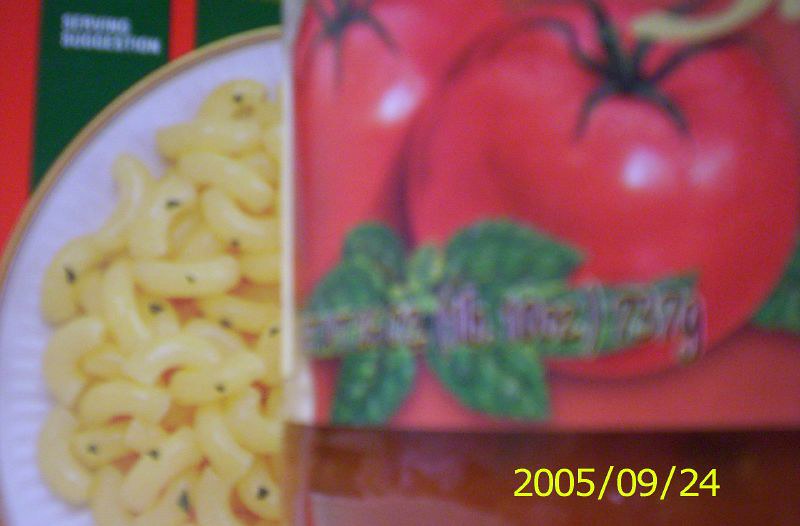This image prominently features a jar of spaghetti sauce, occupying about three-quarters of the frame. The jar is set in sharp focus against a blurred background. The label showcases vibrant red tomatoes still on the vine, accompanied by some green leaves. Information about the product’s weight is visible, along with a date stamped as 2005-09-24. To the side, there is a white bowl or plate containing macaroni noodles, characterized by their yellow hue and a slight black tint. The overall arrangement and details suggest a culinary theme centered around pasta ingredients.